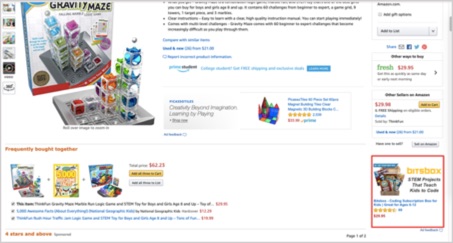The online advertisement showcases the "Gravity Maze" toy game. The cover of the box prominently features a variety of vibrant and intricate structures that can be built using the game components. The premise seems to involve guiding a ball or similar object from the top through a series of interconnected pathways. The pieces are vividly colored in shades of blue, yellow, orange, purple, and a lighter blue, and come in a multitude of shapes, inviting creativity and engineering prowess.

In addition to the box cover, the advertisement displays actual completed structures, highlighting the construction possibilities. Though many words are present on the box, they are too small to be legible in the image. The left side of the advertisement features six thumbnail images, each presumably showcasing different build designs from the game.

The advertisement suggests that additional kits are available for purchase to expand the game further, appealing to those looking to create even more extensive and complex structures. Overall, the Gravity Maze game appears to be an engaging and intellectually stimulating activity, encouraging users to challenge their building and problem-solving skills.